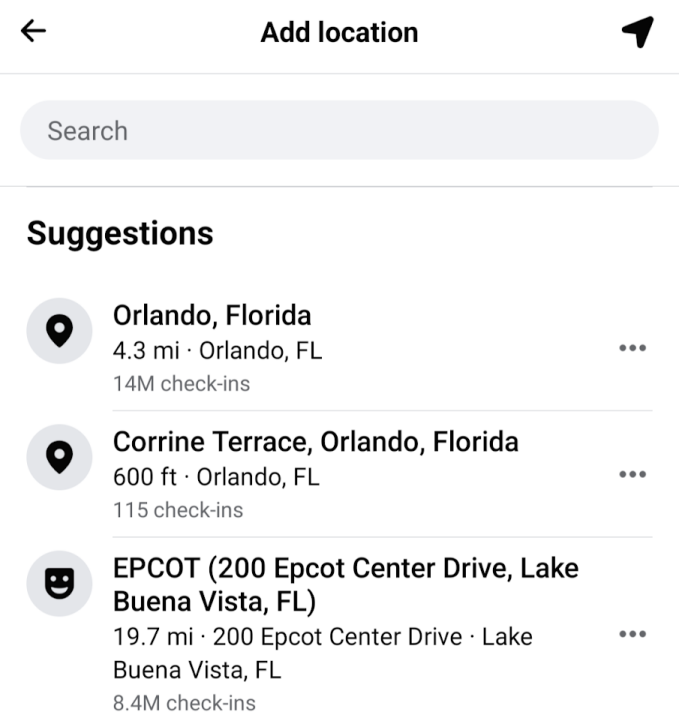A detailed screenshot of a smartphone depicting a location search interface on a white background. At the top, there's a navigation bar with "Add Location" on the left, and a paper plane icon on the right, typically associated with sending messages. Just below, there's a gray search box with the placeholder text "Search," currently empty.

The search interface presents location suggestions:
1. **Orlando, Florida** - 4.3 miles away with 14 million check-ins, followed by three horizontal dots.
2. **Kareem Terrace, Orlando, Florida** - 600 feet away with 115 check-ins, and a row of three horizontal dots.
3. **Epcot** in a gray circle - Detailed as "200 Epcot Center Drive, Lake Buena Vista, Florida," 19.7 miles away with 8.4 million check-ins. This entry also has three horizontal dots to the right.

The overall screen portrays a well-organized location selection interface, offering users quick suggestions for frequently visited or notable areas, complete with distance and check-in statistics, enhancing the user experience for finding and selecting locations.